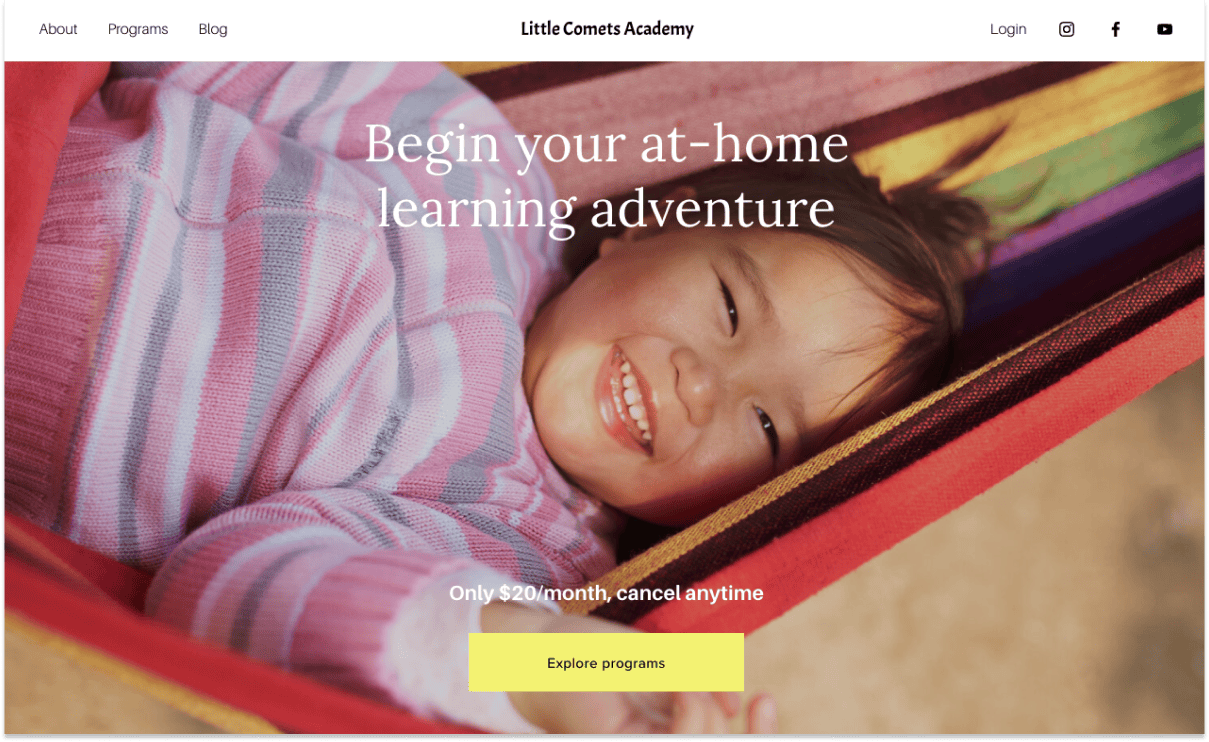The homepage of the Little Comets Academy website prominently features a welcoming visual. At the top center of the page, the "Little Comets Academy" logo is displayed in tiny font against a white background, ensuring it stands out. The navigation menu on the left includes options for "About," "Programs," and "Blog," while the right side features links for "Login," and social media icons for Instagram, Facebook, and YouTube.

Dominating the page is a heartwarming image of a little girl lying in a vibrantly striped hammock, smiling warmly and looking straight at the viewer. She is dressed in a long-sleeve sweater in shades of pink, gray, and white. The hammock itself is adorned with stripes of red, purple, green, yellow, and black. Overlaid on this joyful image, white text encourages visitors to "Begin your at-home learning adventure," with a subtitle offering a subscription for "only $20/month, cancel any time." Just below this message, a prominent yellow button invites visitors to "Explore Programs" in bold black font.

The design elements are minimalistic yet effective, with tan corners at the bottom of the page providing a subtle background. The girl featured is light-skinned with brown hair, red lips, and a bright white smile. Overall, the site is visually inviting and easy to navigate, clearly focused on offering a positive and engaging educational experience for children.